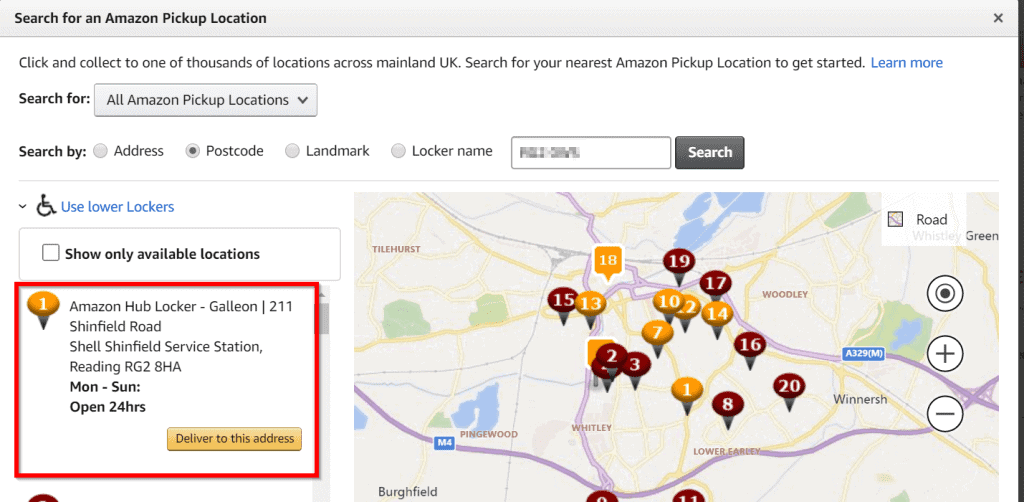The screenshot shows a printout of an Amazon account page detailing the process of finding and selecting a pickup location. At the top-left corner, it says "Search for an Amazon pickup location." Below that, the text reads, "Click and collect to one of thousands of locations across mainland UK. Search for your nearest Amazon pickup location to get started." The phrase "Learn more" is highlighted in blue.

Next, there's a text field indicating that someone has selected all Amazon pickup locations. Below it, left to right, there are labels for "Search, address, postcode, landmark, locker name," followed by a search bar and a search button. The "postcode" option is marked with a dot. Further down, there's a blue highlighted phrase "Use lower lockers" accompanied by a handicapped logo. The option "Show only available locations" is displayed with its checkbox unselected.

In the subsequent section, there's a red-bordered box marked with the number one in white text inside an orange circle. To its right, the details of an Amazon Hub Locker location are provided: "Amazon Hub Locker, Galleon 211, Shenfield Road, Shell, Shenfield Service Station, Reading RG28HA," which is available 24 hours from Monday to Sunday. Below this information, there is a gold bar with black writing that states "Deliver to this address."

Adjacent to this bar on the right side, there's a map showing several numbered locations. The map details areas such as Tilehurst, Woodley, Wintershire, Pengewood, Whitley, Lower Cardee, and Burfield. The indicators for these areas are color-coded in orange and dark burgundy.